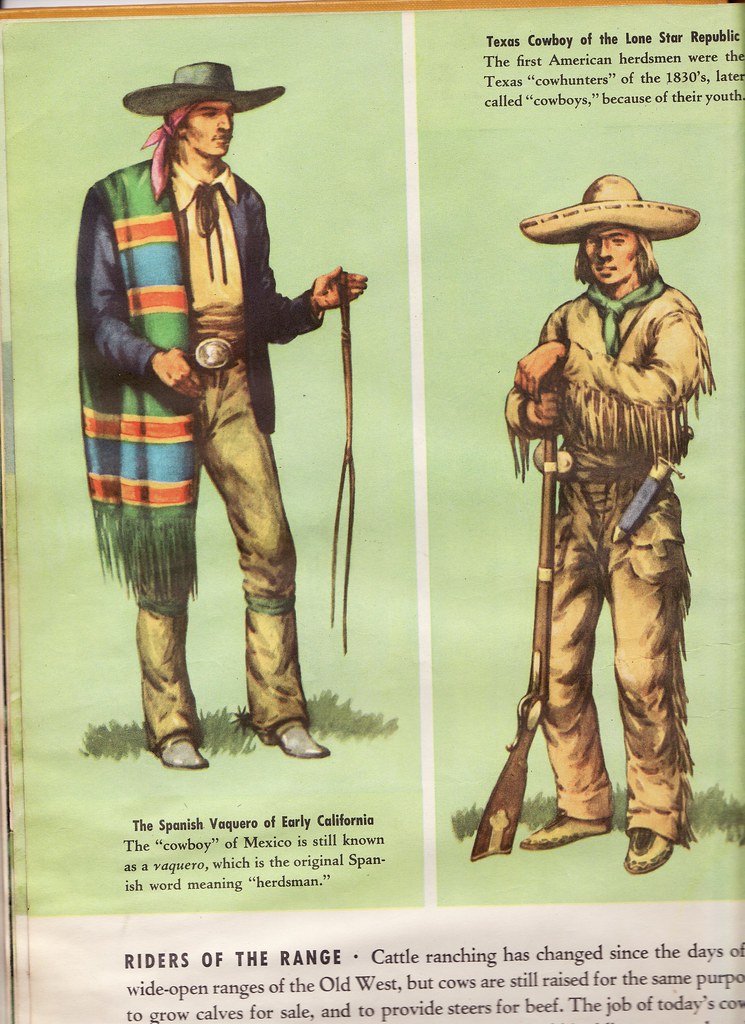This image appears to be a historical illustration sourced from a newspaper or vintage magazine, primarily featuring a green background. The composition is divided into two main sections. On the left, there is an image labeled "The Spanish Vaquero of early California." This figure is depicted wearing a colorful long vest that features green, red, yellow, white, and blue colors, draped over his right shoulder like a poncho. He also wears a green cowboy hat, blue jacket, beige shirt, and beige pants. Notably, he holds a whip in his left hand, and his right hand is tucked into his belt, suggesting a sense of readiness. His attire and posture are emblematic of the early Mexican cowboys, known as Vaqueros—derived from the Spanish word for herdsman.

On the right side, the illustration is labeled "Texas Cowboy, the Lone Star Republic." This character is clad entirely in beige, save for a green tie around his neck, and is wearing a cowboy hat and fringed jacket with cowboy pants. He carries a long shotgun and a knife at his side, suggesting his preparedness for the rugged lifestyle of the 1830s Texas cowboys, who were known as the first American herdsmen. Text accompanying the image mentions that these Texas cow hunters, originally herdsmen in the early 1800s, were later called cowboys, emphasizing their youthful beginnings.

The overall theme of the image contrasts and compares the attire and tools of two distinct types of cowboys—the Spanish Vaquero and the Texas Cowboy, highlighting their roles in early cattle ranching. At the bottom of the illustration, partly cut-off text reads "Riders of the Range, cattle ranching has changed since the days of," pointing to the historical evolution of cowboy culture.